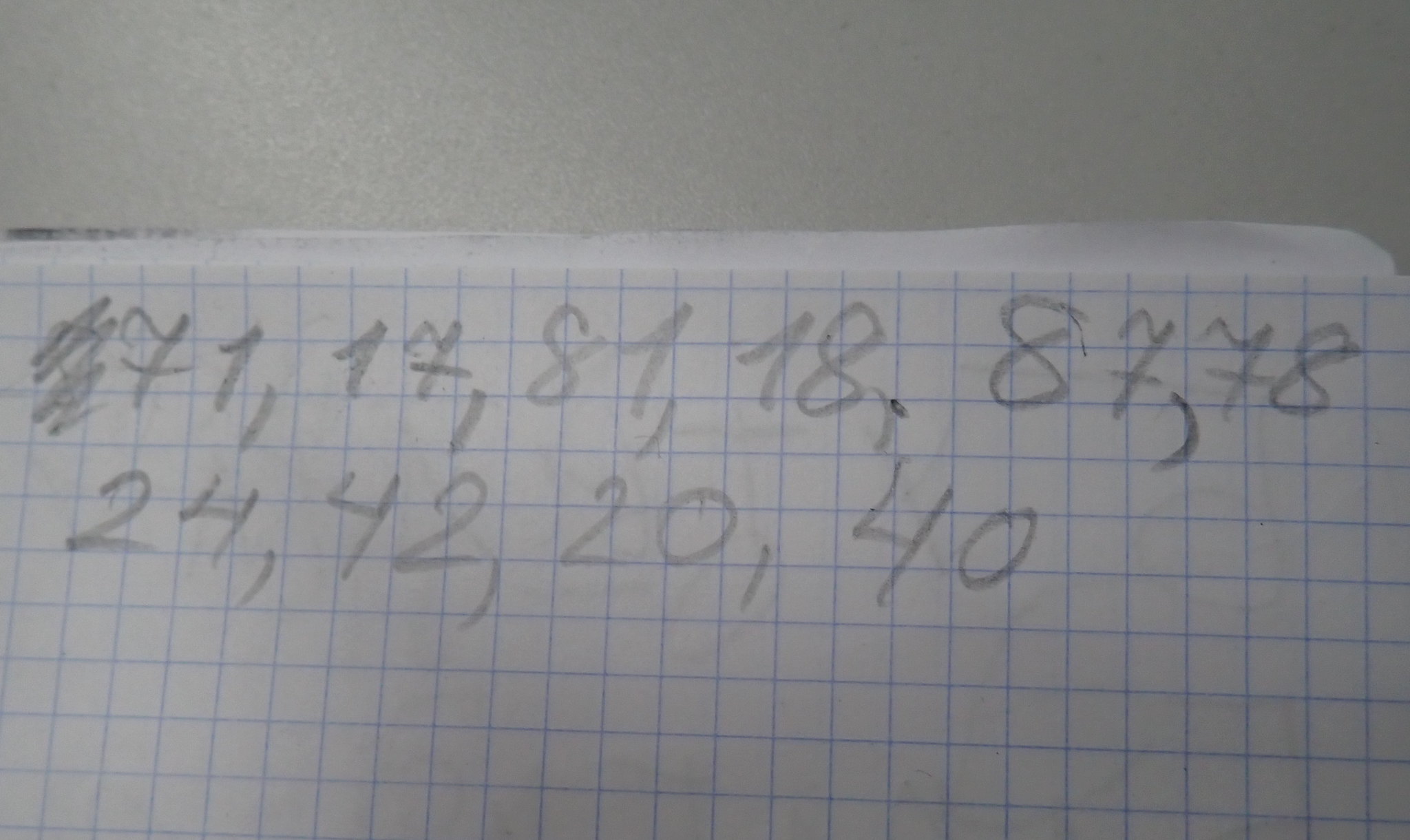A detailed close-up photograph captures a sheet of engineering quadrant paper dominating two-thirds of the image, stretching from the left edge to the bottom edge of the frame. The lines of the quadrant paper are a light blue color. In pencil, a series of numbers are written in two rows. The top row includes a squiggle line, followed by the numbers 71, 17, 81, 18, 87, and 78. The second row beneath features the numbers 24, 42, 20, and 40. The distinctive handwriting includes horizontal hashes through the sevens and notably large commas between the numbers. 

The upper portion of the image reveals a small part of the surface the paper rests on, possibly a white table or countertop. Additionally, a regular piece of paper intrudes into the frame from the upper edge, overlapping the quadrant paper slightly and displaying a slight dog-ear at the upper right corner. 

The photograph is in focus but poorly lit, with a pronounced darker area towards the lower and right side of the image. These lighting conditions give it a somewhat dim ambiance. There are no other visible words, text, or markings on the paper, emphasizing the simplicity of the scene: meticulously penciled numbers on a lightly gridded background.